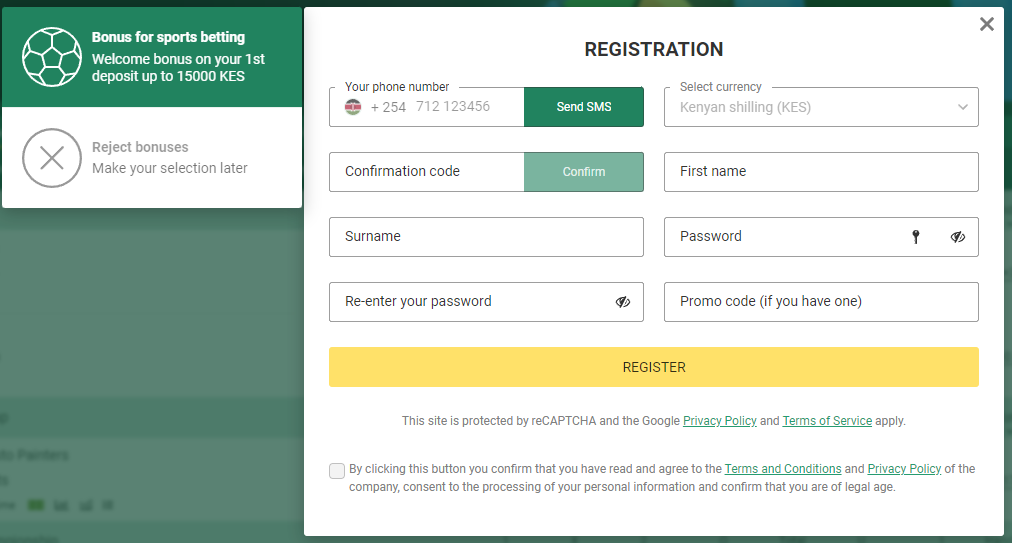The image is a horizontally oriented rectangle featuring a complex layout designed for a sports betting registration interface. The top section is bordered by a dark green or black band, transitioning into a green border that runs down the right side and across two-thirds of the bottom. A thin green strip extends down the left side, covering one-third of the vertical space.

Inside the upper third of the image, a darker green horizontal rectangle features the word "BONUS" in large, all-caps white font, followed by "for sports betting. Welcome bonus on your first deposit up to 15,000 KES" in bold white letters. Adjacent to this text, on the left, is an image of a white soccer ball. Below this rectangle is a white horizontal rectangle displaying a grey circle with an 'X' inside, flanked by the text "Reject bonuses, make your selection later."

The remaining two-thirds of the image has a white background and is focused on the registration process. At the top is the word "Registration" in black text. Below it, there are several horizontal rectangular entry fields:

1. **Phone number**: On the left, an entry box for the phone number, followed by a green button with "Send an SMS" in white text.
2. **Select currency**: Located next to the phone number field.

Next, there are fields for:

- **Confirmation code**
- **First name**
- **Surname**
- **Password**
- **Re-enter your password**
- **Promo code (if you have one)**

Below these fields, a yellow horizontal rectangle features the word "Register" in black text. Further below, in green text, the image states that the site is protected by reCAPTCHA and the Google Privacy Policy, with the terms of service also applying.

At the very bottom, a small square contains a disclaimer in fine print. This text reads: "By clicking this button, you confirm that you have read and agreed to the terms and conditions and privacy policy," with the terms "terms and conditions" and "privacy policy" highlighted in green. The disclaimer concludes by acknowledging the user's consent to the processing of personal information and confirmation of legal age, with the company's consent written in black.